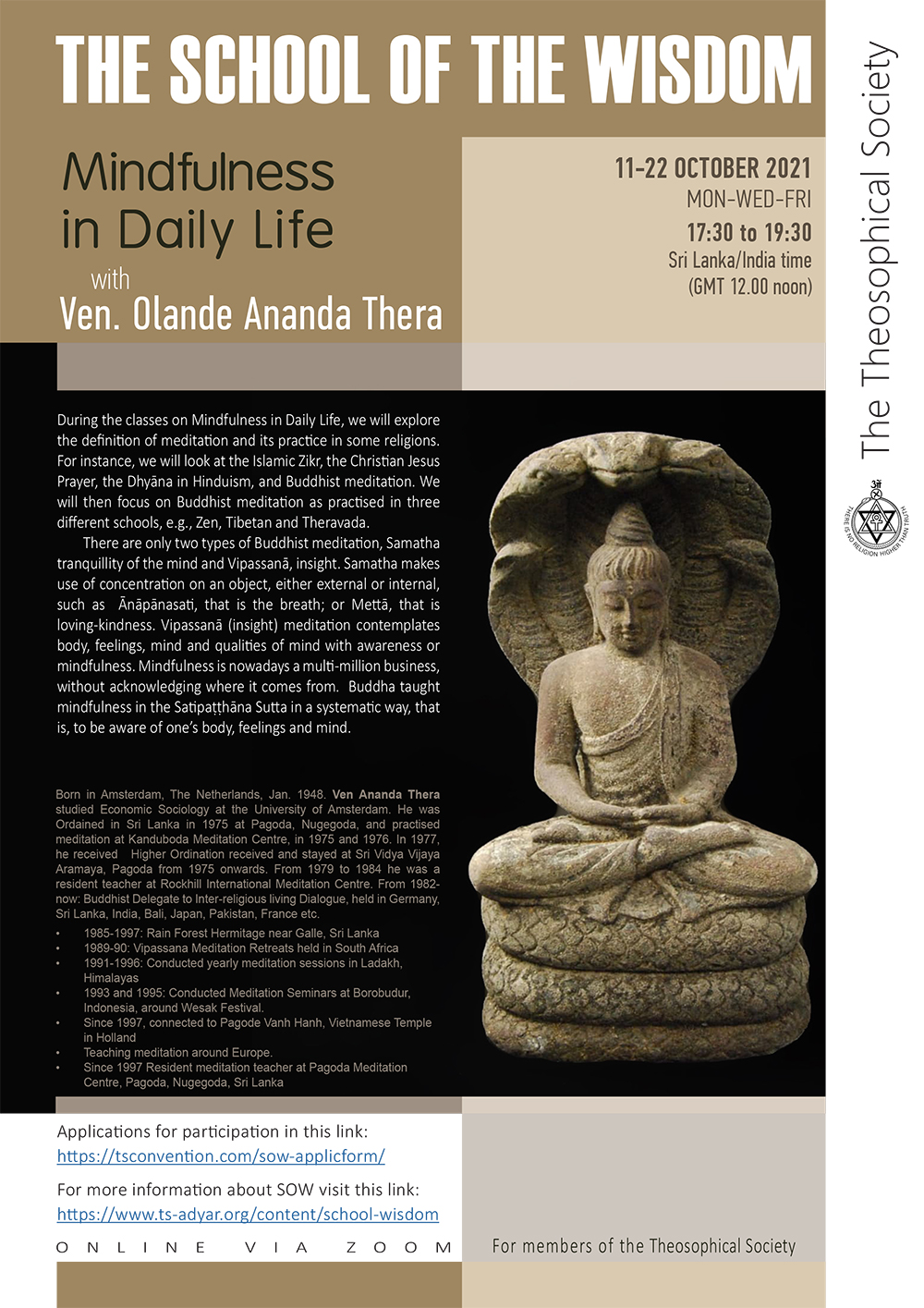The poster is a vertical rectangular format, taller than it is wide, set against a mixed brown and black background. At the top, it features the title "School of Wisdom: Mindfulness in Daily Life" in white text against brown, followed by "with Venerable Olande Ananda Thera" in black text. The event details are provided as "October 11-22, 2021, Monday, Wednesday, Friday, 17:30-19:30 Sri Lanka/India Time, GMT 12 noon."

Below this, the poster includes a descriptive paragraph outlining the class content: "During the classes on Mindfulness in Daily Life, we will explore the definition of meditation and its practice in various religions, including Islamic Zikr, the Christian Jesus Prayer, Hindu Dhyana, and Buddhist meditation. The focus will then turn to Buddhist meditation in Zen, Tibetan, and Theravada schools, highlighting two types: Samatha (Tranquility of the Mind) and Vipassana (Insight)."

To the right of the text is an image of an Indian goddess statue, seated cross-legged on three cushions with five cobra snakes arching over her head. Below the goddess statue is a smaller depiction of a Buddha in a meditation pose, also shielded by five snakes.

The bottom section of the poster includes additional logistical information, such as how to attend the event online via Zoom, and a reference to the Theosophical Society, whose name appears in a black-on-white vertical logo to the right.